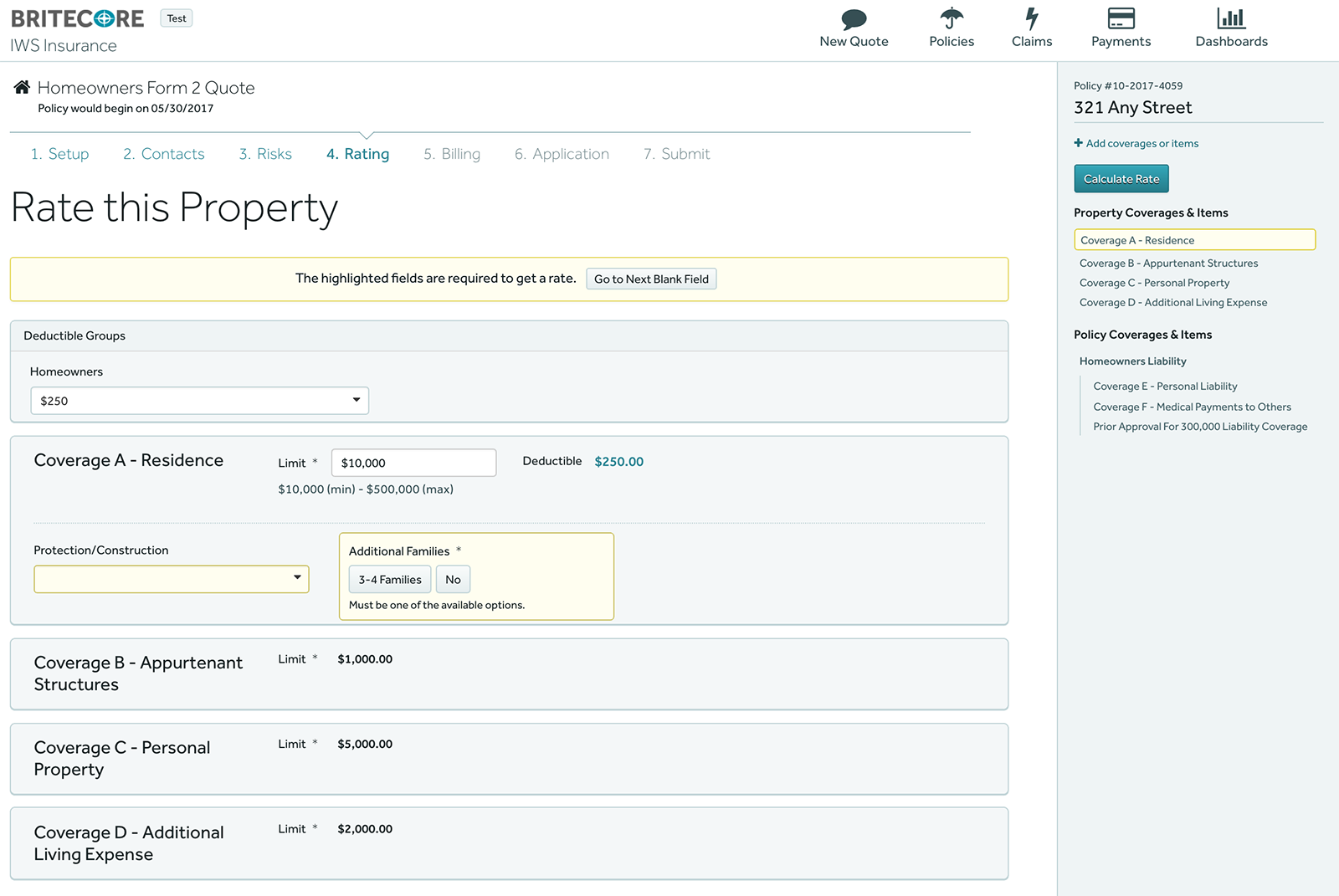This is a highly detailed screenshot of the BRIGHTCORE insurance platform interface. In the upper left-hand corner, the black text spells out "BRITECORE," with "O" stylized as a blue circle featuring a white plus sign. On the upper right segment of the screen are several icons for different functionalities: new quotes, policies, claims, payments, and dashboard.

Beneath the icon row, you'll find a labeled section on the left reading "Homeowners Form," followed by "Quote 2," with some smaller black text underneath whose details are unreadable. A horizontal menu bar runs across the screen, numbered 1 through 7, listing categories such as Set Up, Contacts, Risks, Ratings, Billing, Application, and Submit.

Below this, in prominent black letters, is the prompt "Rate This Property." Directly beneath it lies a horizontal white-brown box with smaller black writing.

On the lower part of the screen, there's a form consisting of multiple sections with a blue background. The right-hand side features a vertical rectangle with a light green background, captioned "321 Any Street" at the top. Smaller text beneath this suggests interactive options for navigating to specific information.

The form at the bottom addresses various coverage options, listed in descending order: 
1. Coverage A - Residents
2. Coverage B - Appurtenant Structures
3. Coverage C - Personal Property
4. Coverage D - Additional Living Expenses